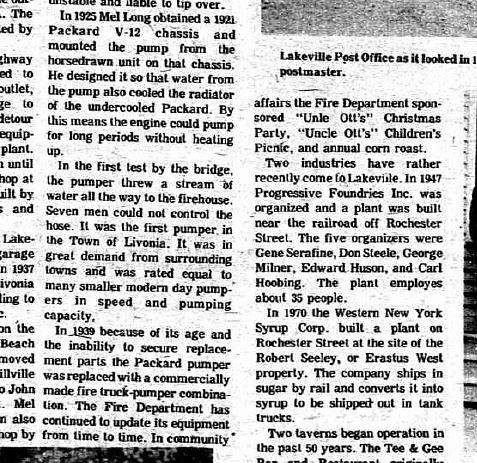The image is a black-and-white close-up of a vintage newspaper article, prominently displaying three distinct columns of densely packed text, albeit without the headline. The upper right portion of the image features a photograph captioned "Lakeville Post Office as it looked in," with the following year obscured. The photograph is only partially visible. The first column reveals a historical narrative from 1925, describing how Mellong innovatively mounted a pump from a horse-drawn unit onto a 1921 Packard V-12 chassis, which revolutionized water cooling for prolonged use. Another segment detailing the fire department's engagements lists several events they sponsored, such as the construction of the Western New York Syrup Corp.'s plant in 1970 on Rochester Street, which succeeded notable local properties. The article depicts the evolution of local services and infrastructure, tying them back to specific innovations and community enhancements.